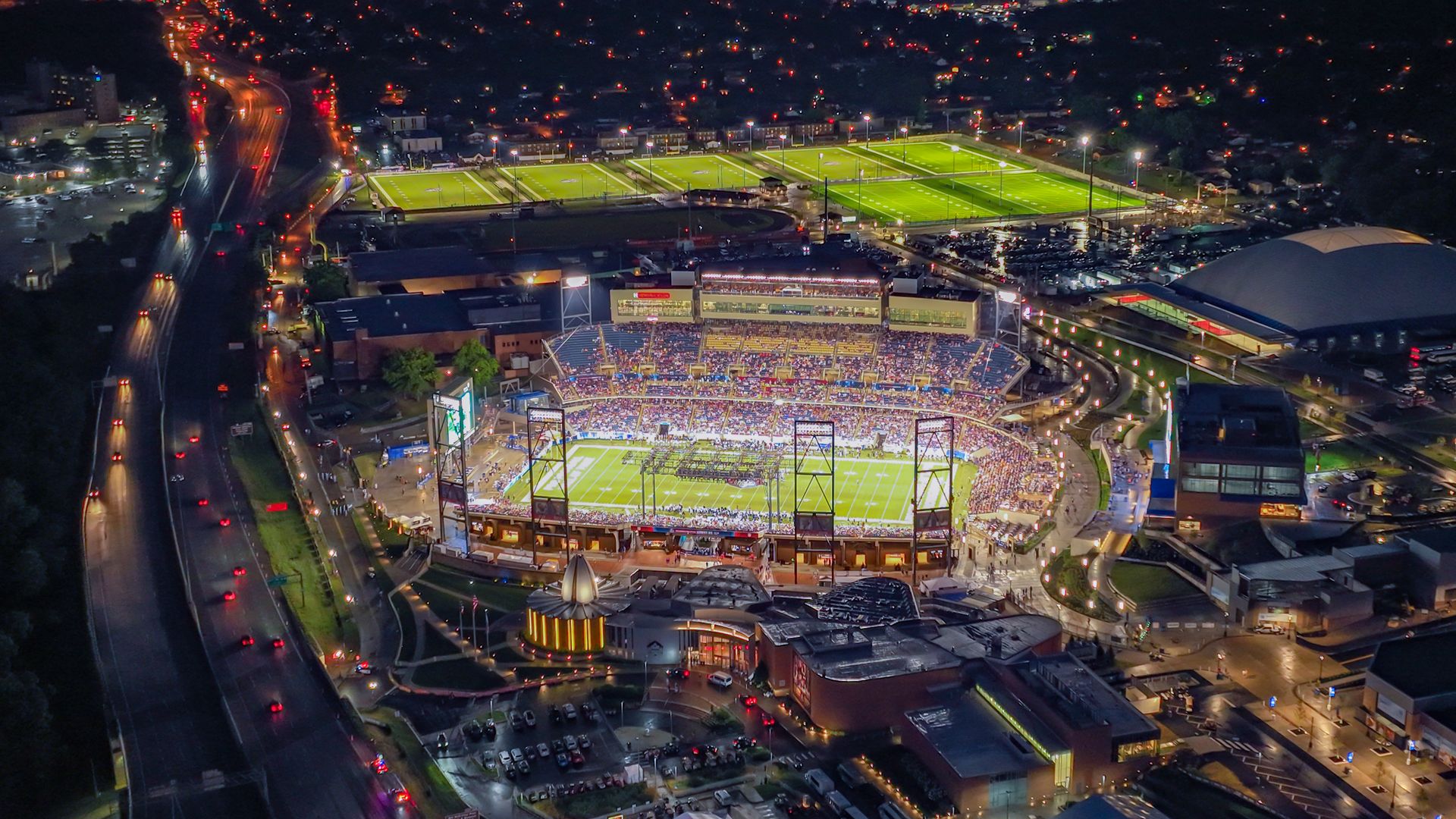This detailed nighttime aerial illustration captures a vast sports complex within a city, dominated by a large open-air stadium surrounded by bright stadium lights and packed with a crowd depicted as tiny circles. The green turf on the field stands out, set against the illuminated backdrop of numerous roadways, including highways and streets that converge at the stadium, showcasing a clear entryway for cars. Adjacent to the primary stadium are seven smaller green fields, arranged with five in a line and two in front, with a dome-shaped building visible nearby. The scene is further highlighted by the glowing red and white car lights on the streets and highways, adding to the vivid, visually stunning depiction. The parking lots, buildings, and distant house lights add depth and context to this lively, bustling nighttime cityscape.